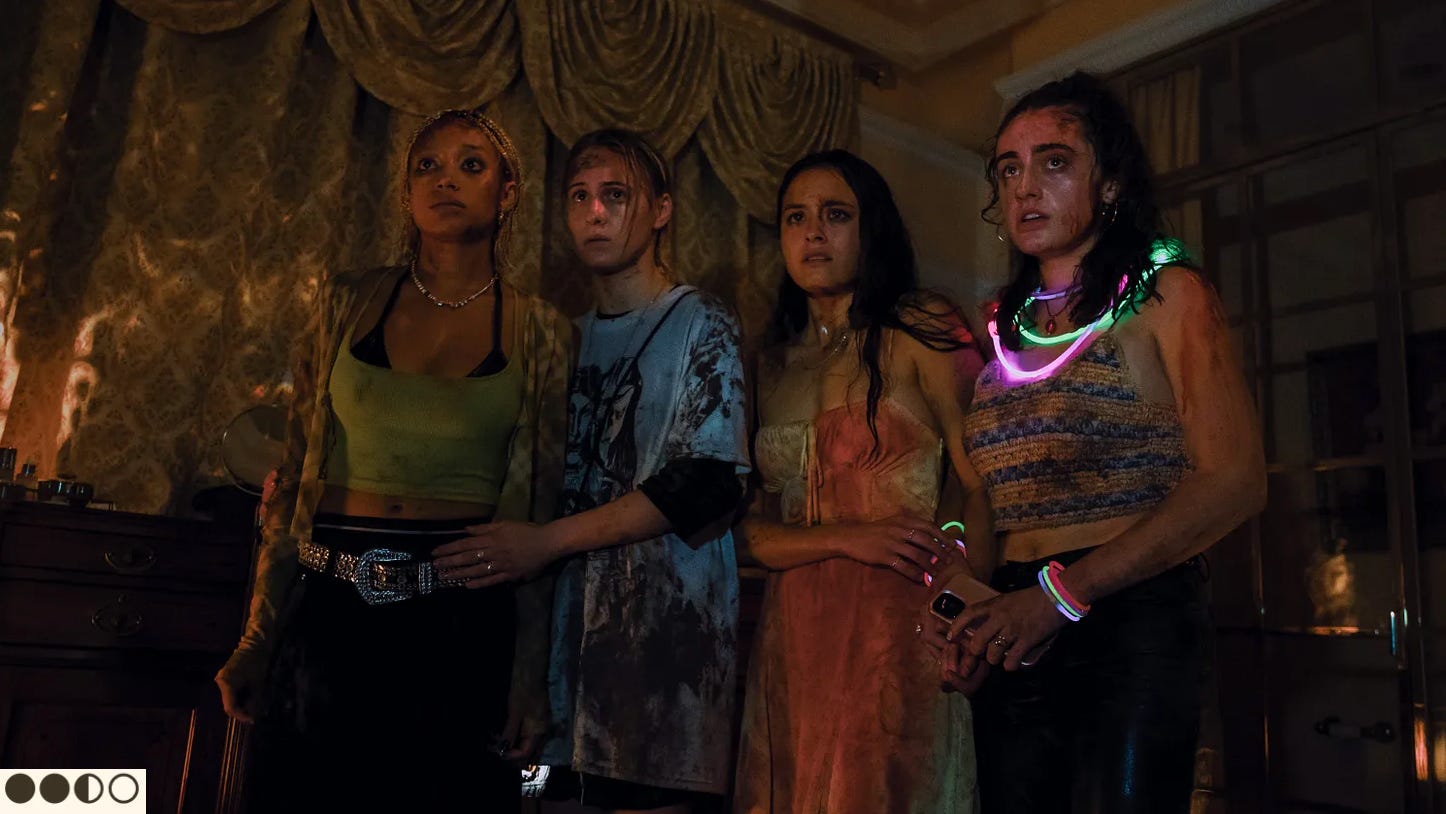This image is a dark and intense scene from the comedy horror film "Bodies, Bodies, Bodies." Four women are at the center of the frame, all appearing terrified and covered in blood, dirt, and sweat. Their attire suggests they were out having fun before finding themselves in this horrifying situation. 

On the left, a girl with black skin wears a green tank top, black pants featuring a prominent belt, and has a bra peeking out. Next to her is a white woman dressed in a blue shirt with black sleeves, embodying a skater-chic look. Another white woman stands out in a blood-stained sundress that was likely once white. Finally, the fourth woman, donning a striped yellow and blue shirt, wears glowing neon necklaces and bracelets reminiscent of a 4th of July parade, highlighting her more festive attire.

All four women are staring in the same direction, visibly scared and repulsed by whatever they are witnessing. They are inside an old, eerie room featuring yellow, brocaded curtains and a piece of wooden furniture. The unsettling atmosphere is amplified by the dim lighting and the reflection of light off the window pane, adding to the creepy ambiance. In the bottom left corner of the image, there are two circles—one filled, one half-filled, and one empty—adding a mysterious element to the chilling scene.